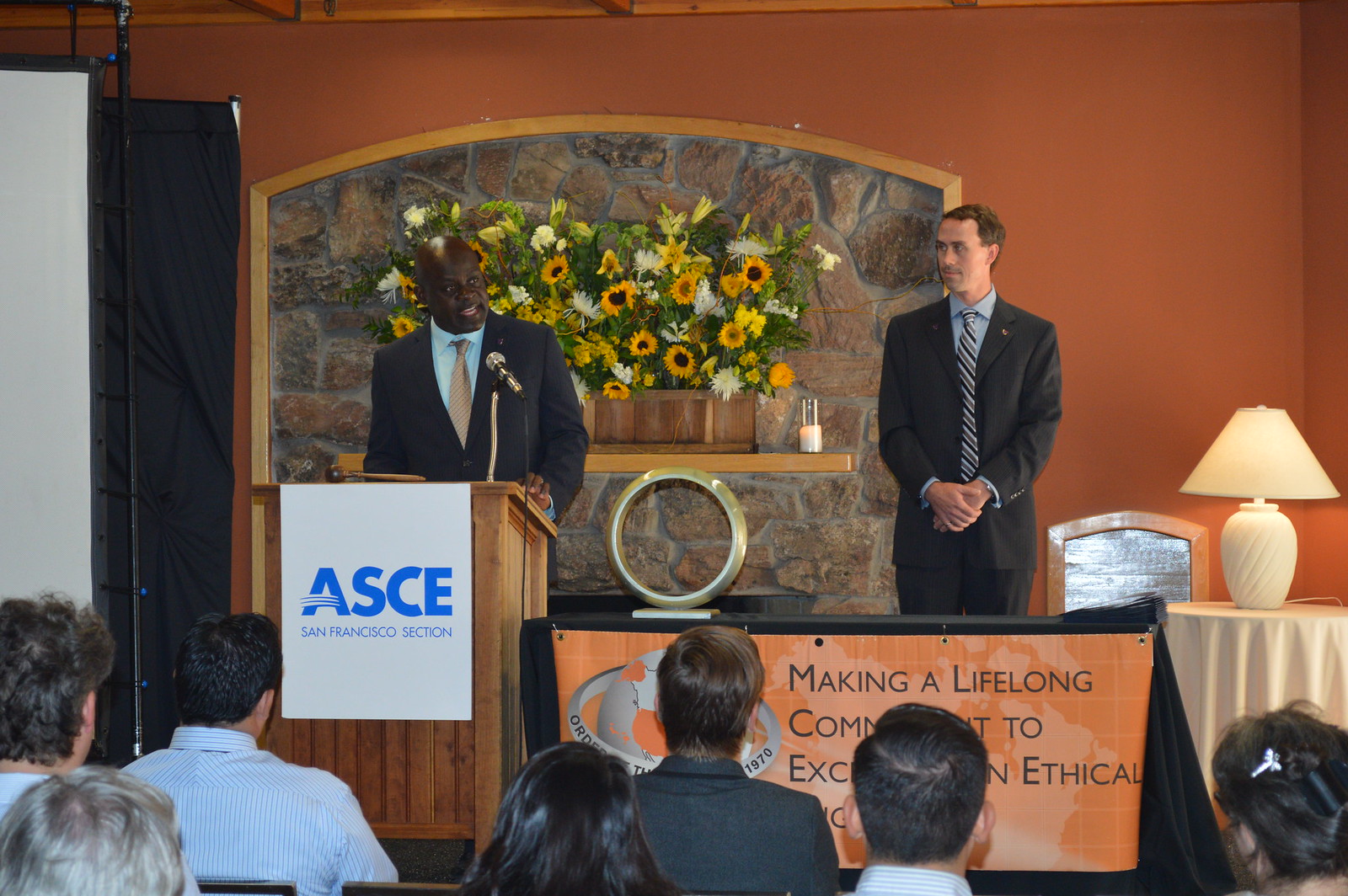This full-color photograph captures an indoor event sponsored by the American Society of Civil Engineers (ASCE), specifically the San Francisco section. At the center of the image, a black gentleman, dressed in a suit jacket, pale blue button-up shirt, and tie, is speaking into a silver microphone from behind a wooden lectern. A sign on the podium confirms the ASCE sponsorship. To his right stands a white gentleman in a suit with a blue striped tie and blue shirt, his hands folded in front of him, attentively watching the speaker. The audience, composed of both men and women, is seated in the foreground, listening intently.

To the side of the white gentleman, there is a small table with a white lamp, and next to it, a chair. Behind them, the wall has a stone recess with an array of flowers, predominantly sunflowers, in a large vase. A large, circular object, possibly an award, is displayed beneath the flowers. An orange banner on a table in the background has text promoting a lifelong commitment to ethical practices. The scene is set against a backdrop of an orange wall, adding warmth to the setting.